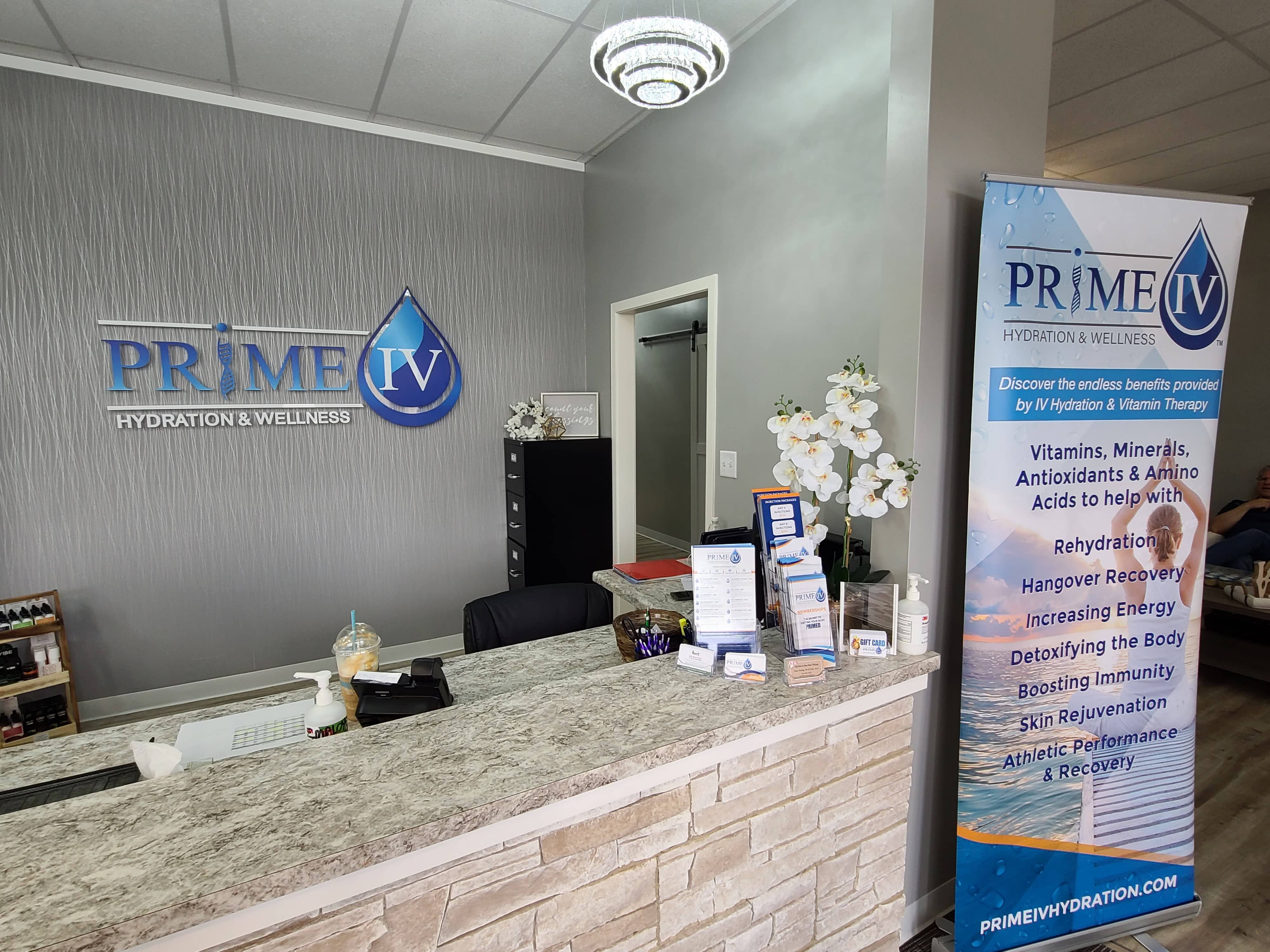This photograph captures the front desk of a Prime IV Hydration and Wellness office, showcasing its elegant stone countertop and matching wainscoting. Prominently featured on the desk are various items, including a computer, a black chair, pamphlets, business cards, a hand sanitizer dispenser, and a small orchid plant. Additionally, there is a cup of coffee or smoothie on the desk. Behind the front desk, the gray back wall, adorned with a texture that resembles cascading water, prominently displays the Prime IV Hydration and Wellness sign, with the "IV" encapsulated in a blue water drop. To the right of the desk, a large advertising poster highlights the benefits of IV hydration and vitamin therapy, featuring a woman performing yoga. The background also reveals a filing cabinet and a shelf stocked with books and extra materials, enhancing the professional ambiance of the medical office.